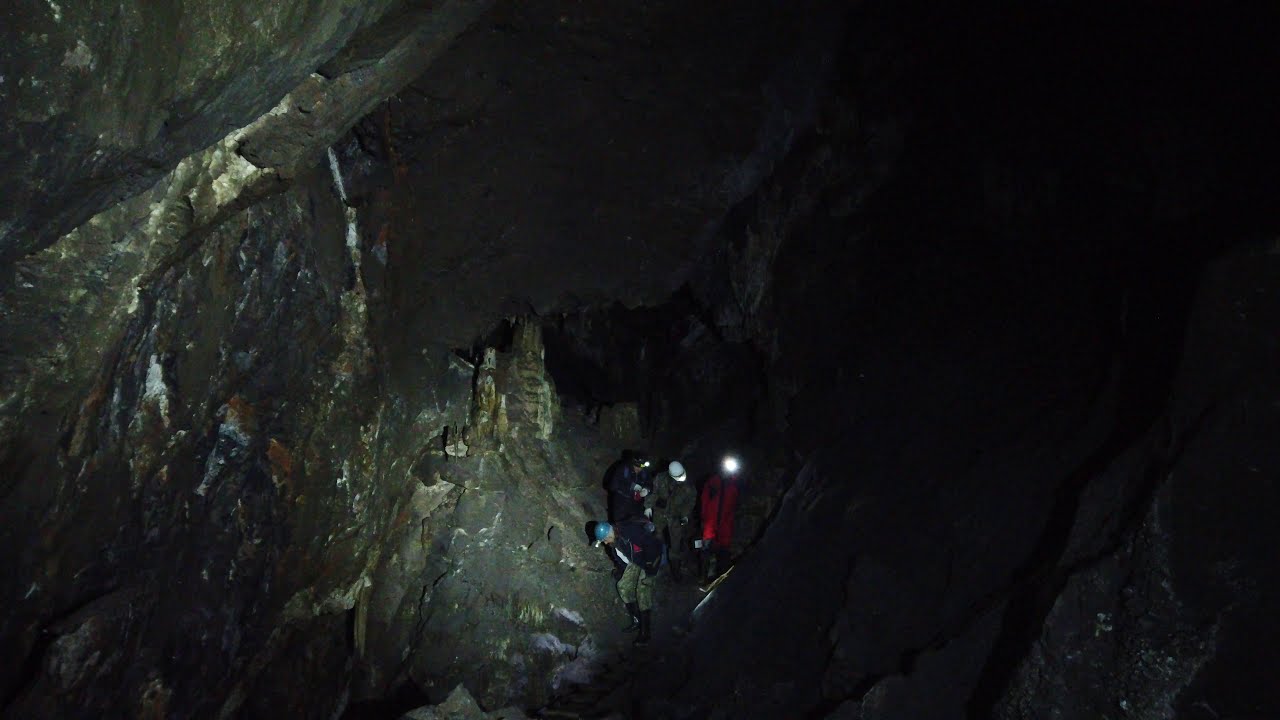The image captures a dimly lit scene inside a cave. On the left side, there are intricate rock formations in dark hues, streaked with patches of light, reflecting natural cave textures in shades of black, gray, and orange. The right side of the image is completely enveloped in darkness. At the center of the photograph, four people are grouped together, their only illumination coming from helmet-mounted lights and a flashlight, as well as the camera flash used to capture this moment. One person is prominently visible in a red jacket and green pants, their helmet light shining directly at the camera, creating a bright glare. To the left of this person stands another individual in dark clothing with their helmet light directed downward to their left. Adjacent to them, another person also dressed in dark attire has their headlamp giving off a faint glow, looking slightly to the left. A fourth person in a blue hat is at the front, bent over at the waist and facing the camera, but looking down towards the ground. The overall ambiance gives a sense of the depth and isolation of the cave, highlighting both the natural cave formations and the careful navigation by the people within.